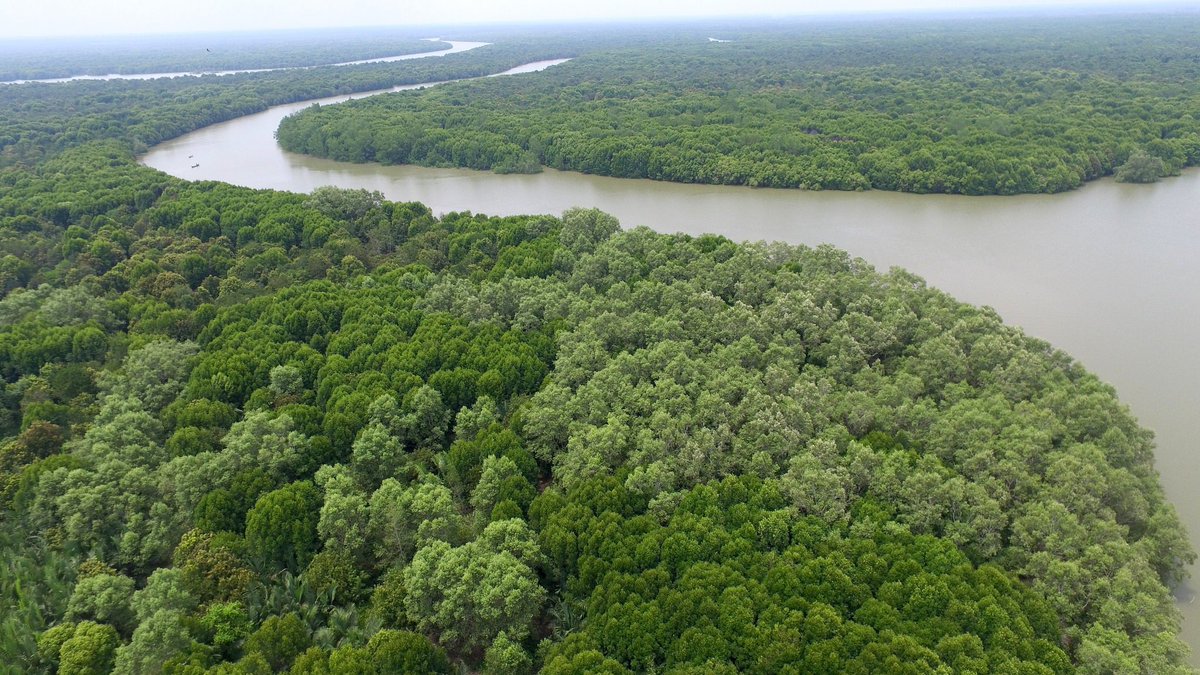This aerial photograph showcases a vast, heavily forested area dominated by hundreds of trees in varying shades of green, from light to medium hues. The dense forest is bisected by a large, winding river that appears muddy, with murky brownish-gray water. Beginning from the middle right side of the image, the river snakes through the thick vegetation, curving multiple times before reaching the upper left corner. Another winding river is faintly visible in the distance. The horizon at the top of the picture is slightly hazy, enhancing the sense of remoteness and isolation in this untouched, humid landscape. No signs of human activity or distinguishing geographical features are evident, contributing to the enigmatic nature of the scene.